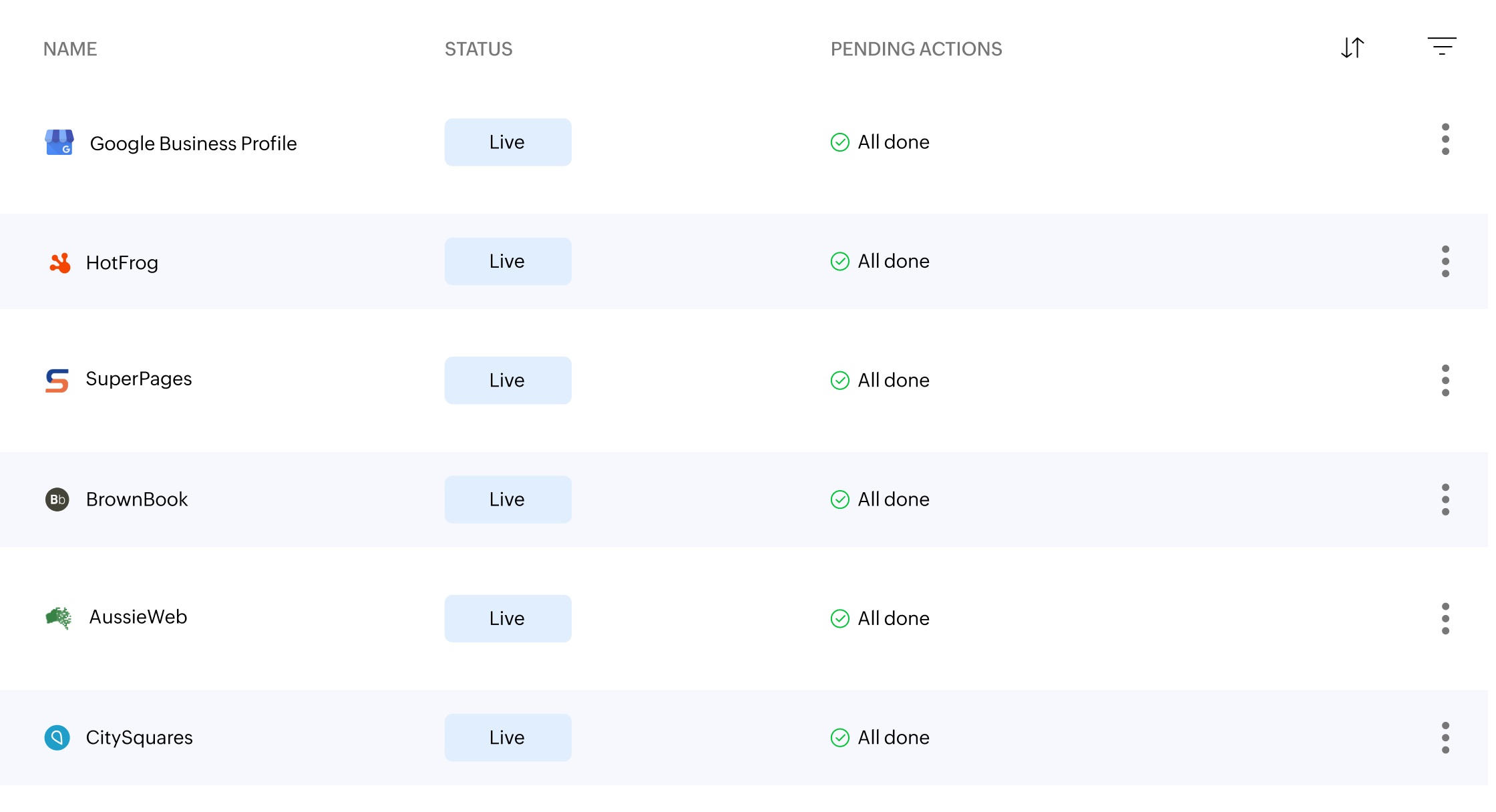This screenshot displays a list of various applications along with their names, statuses, and pending actions. The layout consists of three main columns: Name, Status, and Pending Actions.

1. The **first row** features "Google Business Profile" on a white background. To the left of the name is a blue square with a striped pattern on the top. The status is marked as "Live" within a light blue box, and the pending action shows a green check mark in a circle with the text "All done."

2. The **second row** lists "Hot Frog," identified by an orange frog handprint logo. The background here is light gray with stripes. Similar to the previous row, its status is "Live," and the pending actions are marked as "All done."

3. The **third row** includes "Super Pages," which appears on a white background. The logo is an 'S' with the top half in blue and the bottom half in orange. The status is "Live," and the pending actions display "All done."

4. The **fourth row** contains "Brown Book," displayed with a brown circle logo featuring a capital 'B' overlapping a lowercase 'b,' both in white. The status reads "Live," with "All done" under pending actions.

5. The **fifth row** shows "Aussie Web," distinguished by the green outline of Australia in its logo. It also has a status of "Live" and marks "All done" under pending actions.

6. The **sixth row**, in light gray, lists "City Squares," represented by a blue circle with a white shape inside. This entry is also marked as "Live" and "All done."

Additionally, each row includes a set of three dots on the far right side, potentially for additional options or actions related to the respective applications.